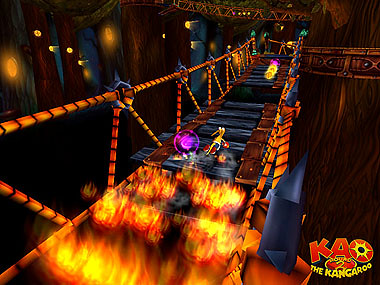A vibrant image resembles a 90s video game scene, showcasing a thrilling moment from the game "KAO: Round 2." In the bottom left corner, the game's red and yellow logo prominently features the word "KAO." Dominating the scene, a kangaroo character with a distinctive purple horn races across a deteriorating and burning bridge. The fire seems to be in the process of consuming the bridge, causing it to disintegrate, adding an intense sense of urgency. The objective is clear: the character must run as fast as possible to avoid plummeting into the abyss. Along the treacherous path, sparkling coins are scattered, waiting to be collected, adding an element of challenge and reward to the high-stakes dash.